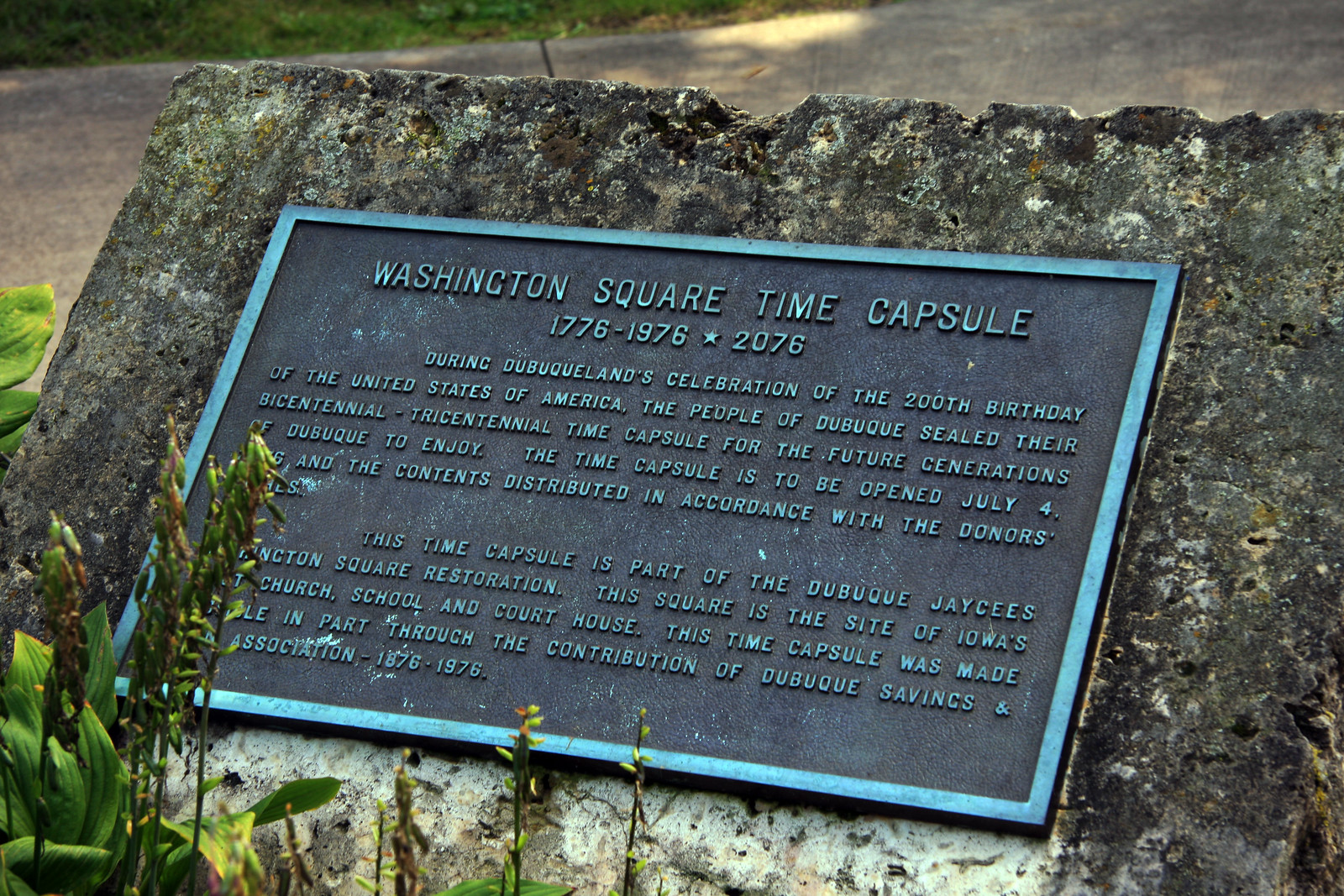The image captures an outdoor setting in a park, showcasing a rectangular black metal plaque with a light blue border. The plaque is mounted on a naturally shaped, aged black and white stone at a 45-degree angle. Positioned amid some plants and grass, with a walkway visible in the background, the plaque reads: "Washington Square Time Capsule, 1776-1976-2076." It commemorates the sealing of Dubuque's Bicentennial Triennial Time Capsule during the celebration of the 200th birthday of the United States, intended for future generations to open on July 4th, 2076. The plaque acknowledges its creation as part of the Dubuque J.C.'s Washington Square restoration, a historic site for Iowa's church, school, and courthouse, made possible through the contribution of Dubuque Savings and Association (1876-1976). Some of the text is partially obscured by plants growing in front of the stone.